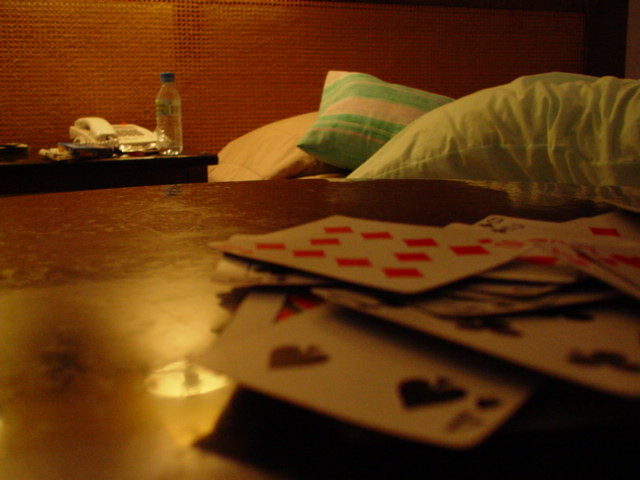In this dimly lit bedroom photo, taken from the top of a brown wooden table, the scene captures a casual and intimate setting. Scattered directly in front of the camera are several playing cards, haphazardly arranged with some face-up; the Ten of Diamonds and Four of Spades are clearly visible among the loosely stacked deck. The table's surface reflects a nearby lamp, suggesting a warm, ambient glow. Across from the table, a nightstand holds a landline phone, a water bottle, and what appears to be a remote control, adding functional details to the room. In the top right of the photo, the bed is visible, adorned with multiple pillows—one green and white, another purely white, and a third green cushion. The wall behind the bed is made up of an unusual pattern of tiny brown squares, contributing to the cozy and distinctive atmosphere. Soft light filters in from above, enhancing the room's tranquil and inviting aura.